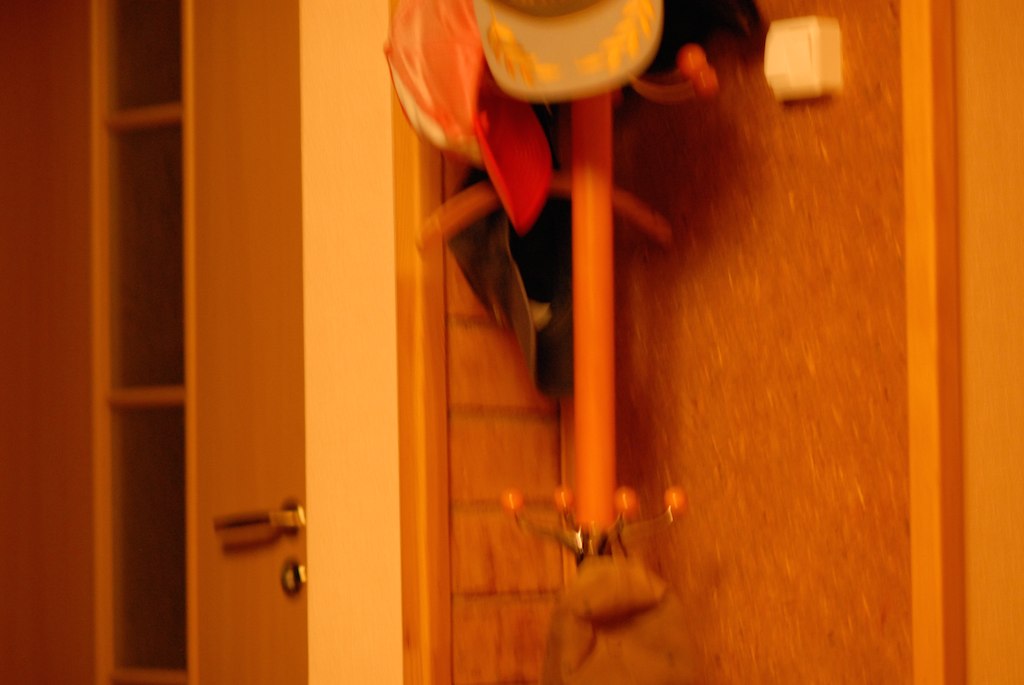This photograph showcases an orange cylindrical coat and hat rack, likely made of plastic. The rack prominently displays two hats: a baseball cap adorned with gold scrambled eggs, and a satin-like bicycle riding hat with an orange sheen and a sun visor. Additionally, the rack features multiple hooks, including one with a cap hanging in the middle. To the side, there is a hanger affixed to what appears to be a thermostat on a wall. The scene reveals part of an empty closet, with wood slats and caulk forming a corkboard wall, painted in a deep cream color. The closet door is also made of wood, contributing to the rustic aesthetic of the space.